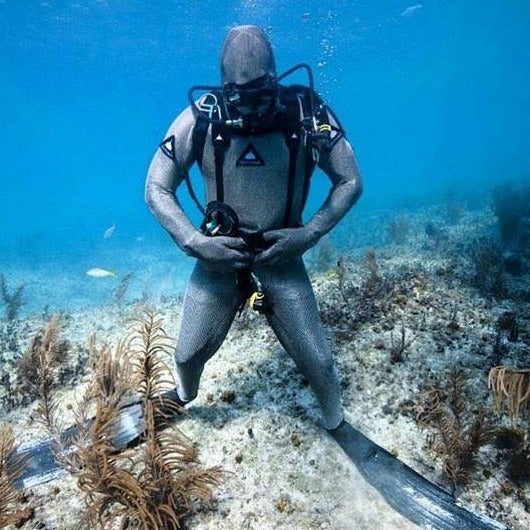This underwater photograph, though somewhat blurry and grainy, features a scuba diver standing on the ocean floor. The diver, dressed in a sleek gray wetsuit and matching flippers, has a breathing apparatus with oxygen tubes in his mouth and black goggles on his face. Bubbles can be seen rising on his right side. His hands are gripping the belt area of his suit, and he appears to be posing for the camera with his knees slightly bent. The ocean floor beneath him is mostly white sand with patches of brown seaweed-like plants scattered around. In the clear, blue water above, two small fish swim near the left side of the image, adding to the serene underwater scene. The photograph captures a calm moment beneath the waves, with the diver as the central focus.